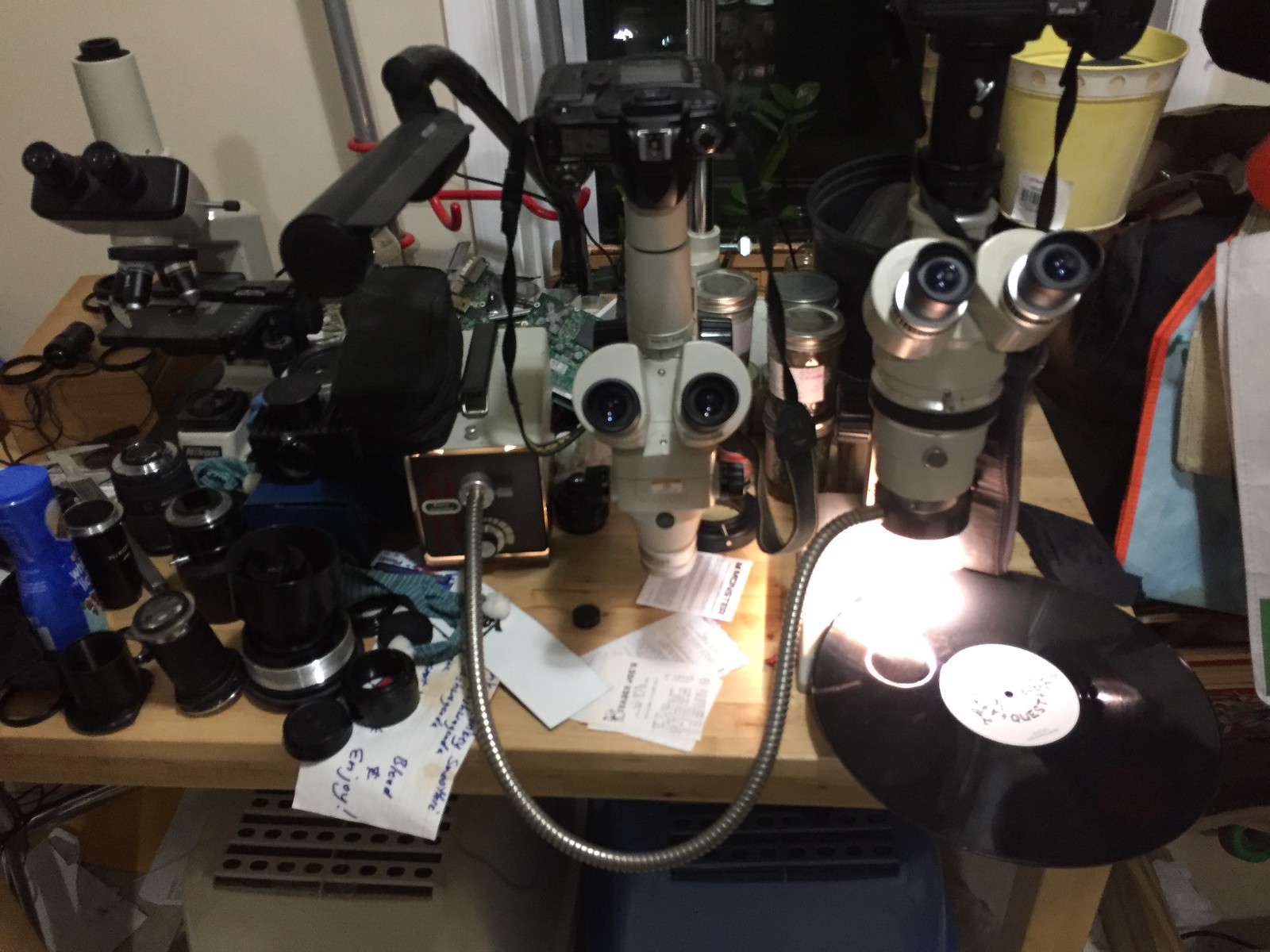The indoor photograph presents a scene of notable disarray centered around a wooden table laden with scientific equipment and miscellaneous items. Dominating the clutter are multiple microscopes—at least three—among which one is powered on, casting light onto a vinyl record positioned below. Scattered papers, both with printed text and handwritten notes, enhance the sense of chaos. Additional scientific paraphernalia includes microscope lenses, a potential spectrometer, and mason jars topped with silver lids. A yellow flower pot, a bright blue spray can, and a black album with a white label add to the eclectic assortment. Beneath the table, there are two plastic animal carriers, one beige and one blue. Also visible is a thick, ridged metal cord linking two devices, alongside what appears to be a camera and a white object with a long silver hole at the forefront. The overall impression is one of clutter and disorganization.